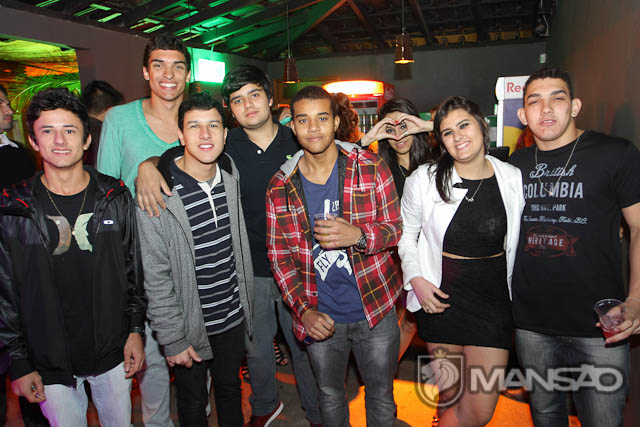The photograph captures a lively group of friends, likely in their 20s, posing together in a vibrant bar or club setting. The atmosphere of the venue is lively, characterized by various bright lights hanging from the ceiling and a neon-lit background, possibly featuring a Red Bull machine. The group consists of six young men and two young women, all with dark brown hair. They are all smiling and seemingly enjoying their time, some holding plastic cups that likely contain alcoholic beverages.

From left to right, the group includes: a guy in light-colored jeans and a black shirt, possibly a Hurley brand; next to him, a guy with black pants and a horizontally striped polo shirt, covered by a gray zip-up hoodie. Behind him is another boy wearing a green t-shirt with a wide neckline. To the right, there is a guy wearing gray pants and a black shirt, followed by a boy in a red plaid jacket over a purple shirt. Slightly behind this last boy is a girl making a heart symbol with her hands—framing her eyes through the shape—wearing a black shirt. Next to her, a girl in a white jacket and a short black skirt, her midriff slightly showing, smiles warmly at the camera. Finally, to the far right, a guy in a black T-shirt with white writing, possibly reading "Columbia," holds a drink in his hand. His dark gray jeans and short, spiky hair complete his look.

At the bottom right corner of the photograph, a logo resembling a shield with a possible lion’s head is overlaid, accompanied by the name "Mansao." The background of the image features a mix of colored lights, casting a fun and energetic aura over the scene.